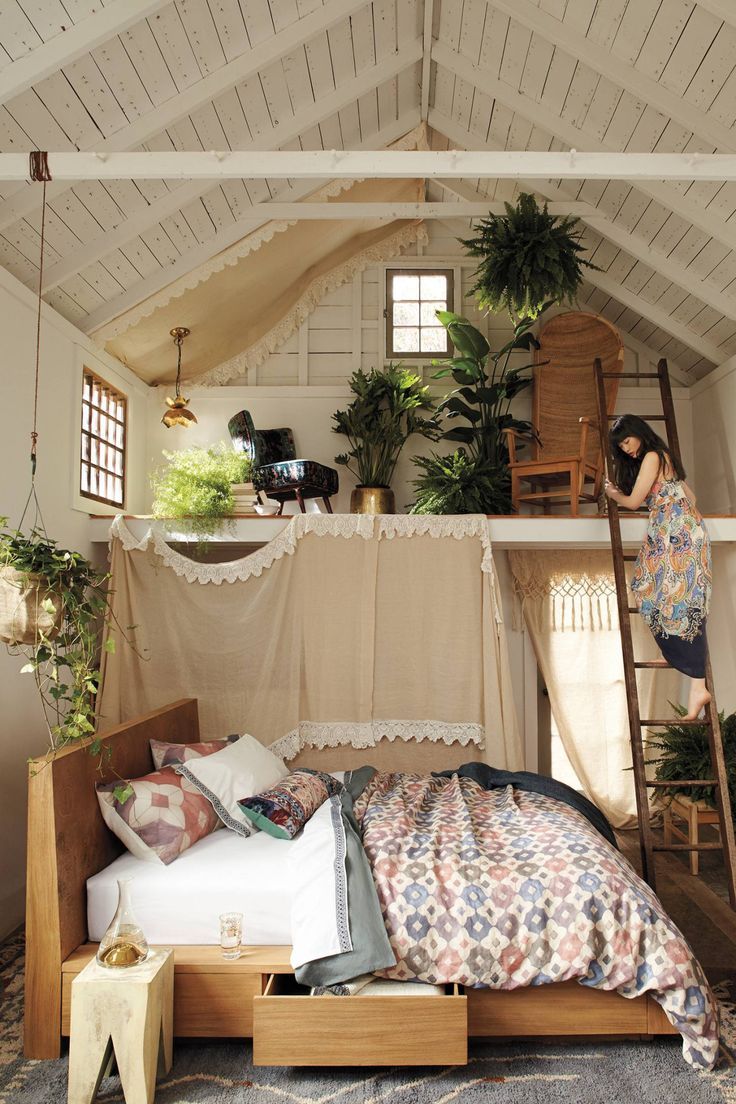This detailed photograph captures the interior of what appears to be a well-decorated tiny house designed with efficient use of vertical space and natural light. Dominating the image is an impressively tall cathedral ceiling that creates an airy atmosphere within the small structure. In the foreground, there's a platform bed dressed with white sheets, pillows, and pretty linens, featuring built-in drawers for storage. Adjacent to the bed is an artsy, contemporary night table crafted from light wood with animal-like legs.

An array of plants, including hanging and potted varieties, bring a touch of nature indoors and add to the cozy, inviting ambiance. To the right of the bed, a draped area suggests a separate space, likely for added privacy, complemented by another drape over a window nearby.

A central element is a wooden ladder positioned on the right, leading up to a loft area where an Asian woman is seen climbing down. This loft, illuminated by ample natural light from the windows, serves as a seating or reading nook, evident from the presence of chairs and a stack of books. The white-painted wooden interior and multiple plants, including ferns, contribute to the serene, aesthetically pleasing environment of this charming, multifunctional living space.